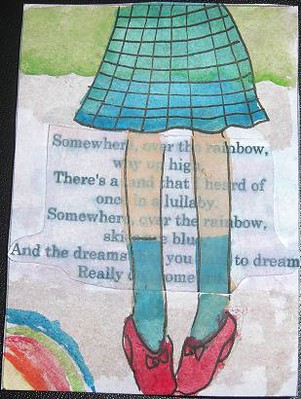This is an illustration resembling a watercolor painting typical of a child's book. Dominating the scene is a blue skirt with a grid pattern, descending from the top of the image. Out from under the skirt extend two legs with a nude pink tone, adorned in long blue socks that match the skirt, and red shoes accented with matching red bows. The background is split into two main colors: green from the middle of the skirt upwards and a creamy white from the middle downwards. 

In the lower left corner, a rainbow displaying shades of blue, green, pink, and red adds a splash of vibrant color. Superimposed behind the legs is partially obscured text, reading, "Somewhere over the rainbow, way up